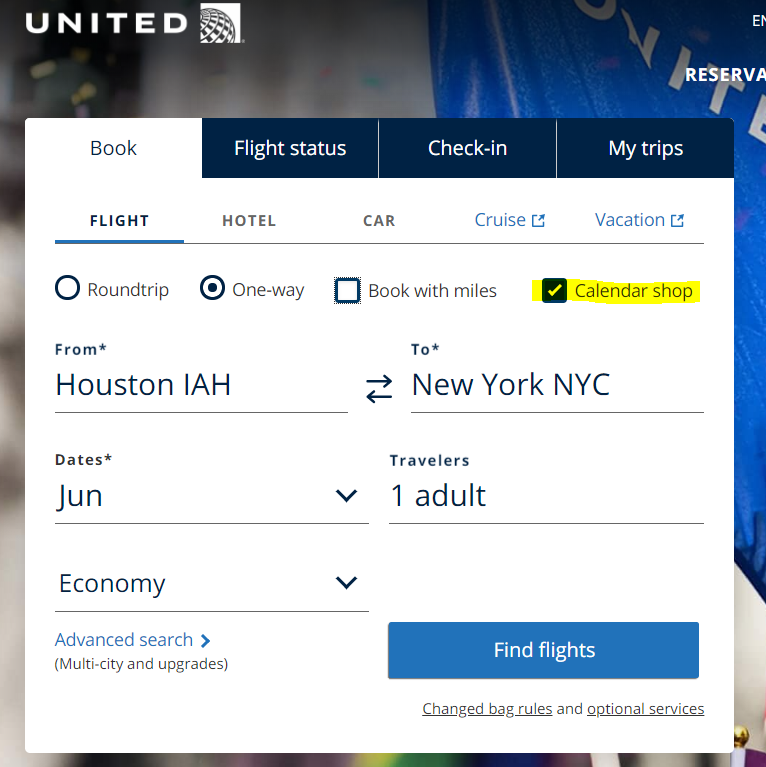**Description:**

The screenshot appears to be taken from the United Airlines website. The background features an abstract representation of the United Airlines flag, which transitions from black on the left to gray and then white on the upper right. The word "United" is faintly visible in white text within the background.

In the top-left corner of the main page, the word "United" is prominently displayed alongside a white circle containing the United globe logo. To the right, partially visible, is the beginning of the word "reservation" which is truncated due to a white pop-up box.

The white pop-up box features the word "book" in blue text, and three blue sections with white text reading "Flight Status," "Check-in," and "My Trips." Below this, a white background contains clickable text options for booking different types of services: "flight" in bold black text underlined in blue, followed by "hotel" and "car" in gray, and "cruise" and "vacation" in blue.

Under the service options, we see two black circles indicating round-trip and one-way options with respective labels. A square labeled "Book with miles" is unchecked, and there is a highlighted yellow option for the "Shop Calendar" which is checked.

Further details include a booking form with fields for departure and arrival locations ("Houston IAH" to "New York NYC"), travel dates in June, the number of travelers (adults), and the travel class, which is selected as "Economy." Below this, blue text offers an "Advanced Search" option, with gray text options for "Multi-city" and "Upgrades."

On the right-hand side, a prominent blue button with white text says "Find Flights," ready to initiate the search process.